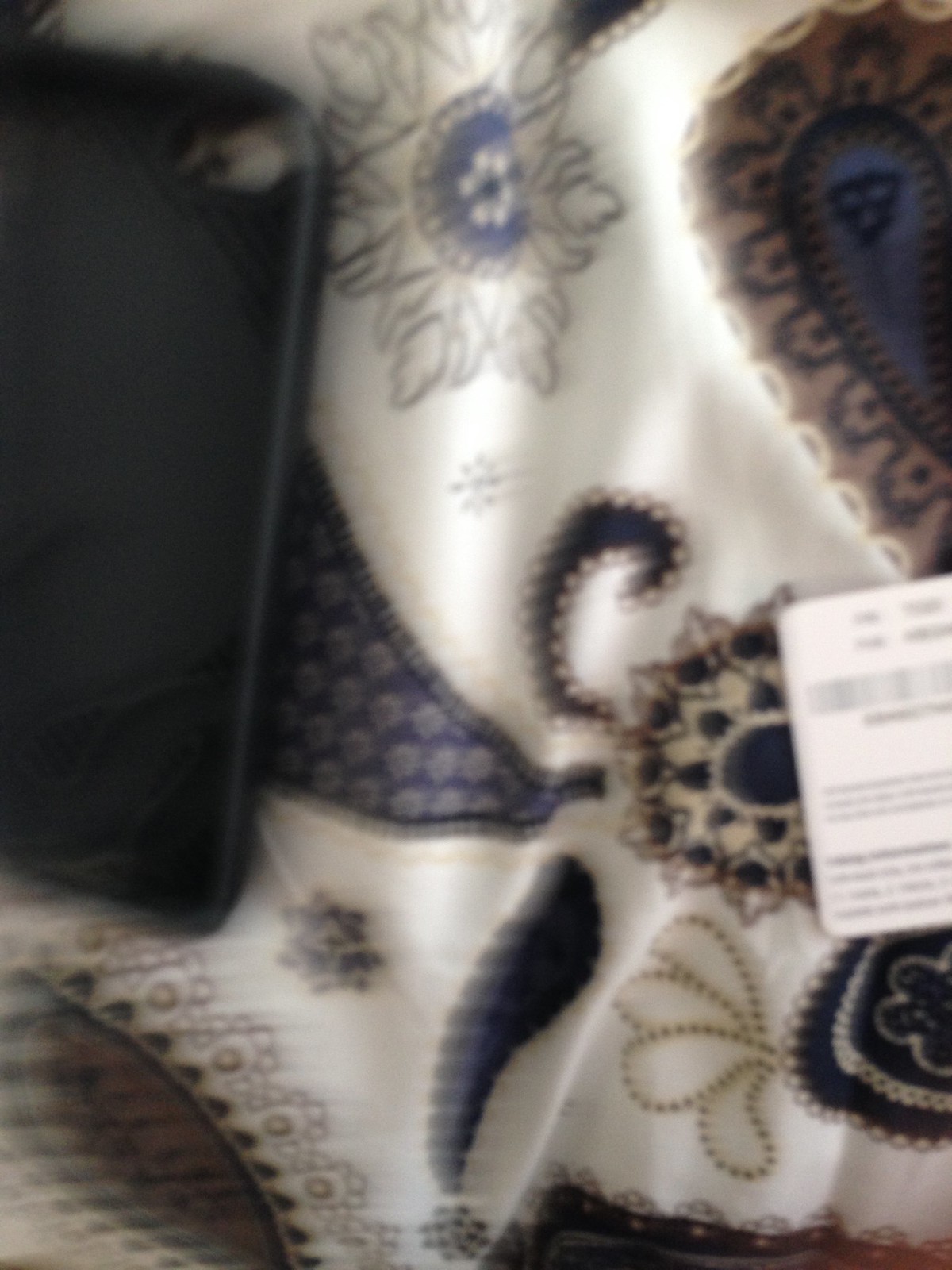This image captures a somewhat blurry close-up of a piece of fabric that appears to be an article of clothing. The fabric in question is a lush, white satiny material adorned with intricate floral patterns in navy blue and cream colors. A store-issued white tag remains attached to the cloth, indicating it is likely a newly purchased item. The cloth is slightly bunched up, adding texture and layers to the visual. In the upper left corner of the frame, a cell phone in standby mode rests atop the fabric, its screen dark and unlit. A subtle gleam of light shines on the white part of the satin, creating a delicate reflection that accentuates the fabric's sheen.